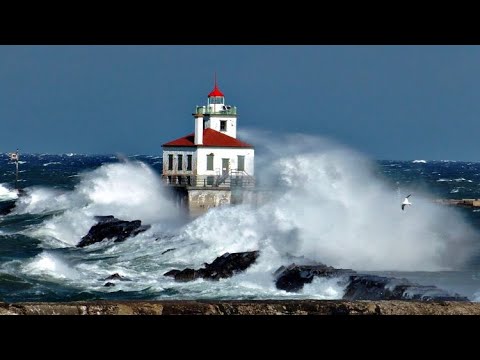This photograph captures a striking scene of a white lighthouse with a red roof, standing resolutely amidst a tumultuous blue ocean. Positioned towards the center of the image, the lighthouse is being relentlessly battered by aggressive waves, which create a dramatic white spray that envelops the building in a misty haze. The sea appears powerful and forceful, crashing into the black, jagged rocks that partially surround the lighthouse and provide some defense against the water's fury. The skyscape is clear and blue, adding to the vivid contrast of the scene. A seagull is visible in the foreground, adding a touch of liveliness to the otherwise human-less scene. The lighthouse, featuring tall rectangular windows and a green door, stands tall and strong against the fierce ocean, symbolizing resilience amid nature’s relentless assault.